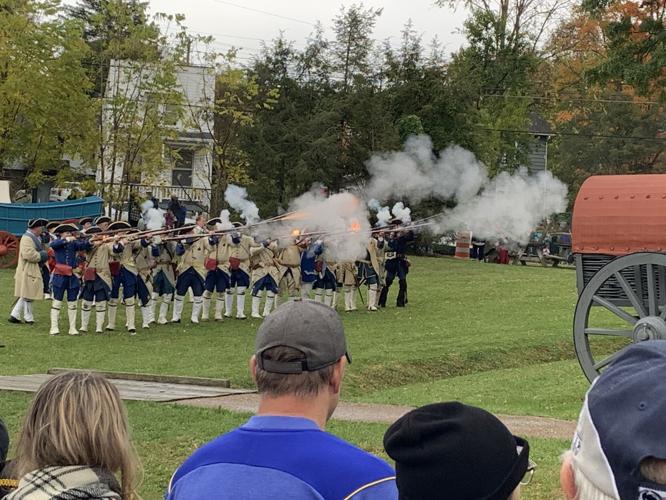This photograph captures a detailed Revolutionary War reenactment scene set in an expansive green field. In the foreground, spectators dressed in contemporary clothing—including one notably in a baseball hat—are seen from behind, attentively watching the historical spectacle. Beyond them, a single file of colonial soldiers, clad primarily in blue uniforms with some wearing tan overcoats, is prominently displayed. With muskets aimed, the soldiers fire in unison, creating dramatic clouds of smoke and visible flames. To the right of this line of reenactors, part of a wagon is noticeable, specifically its wheel and the red top. The background features a small house and tall trees, suggesting a rural setting. The sky is overcast, lending a somber, diffused light to the daytime scene, though the sun itself is not visible.